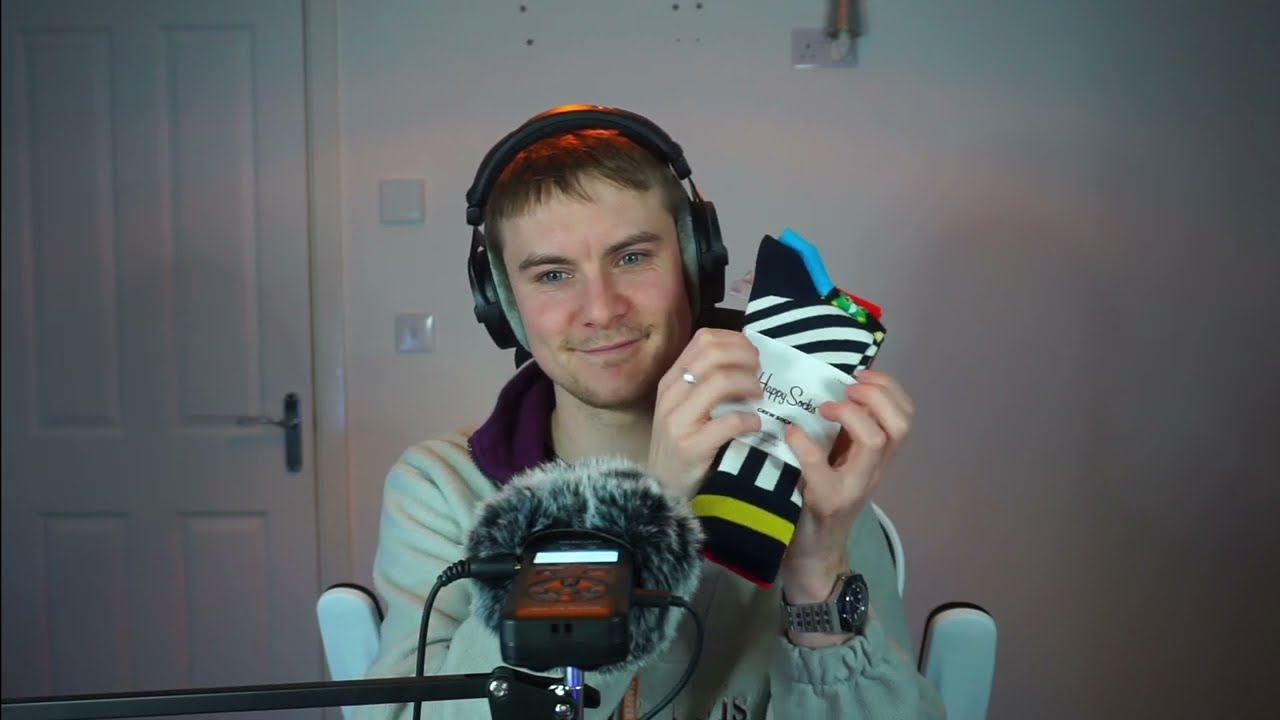In an indoor setting, possibly a bedroom, a man in his mid-30s sits in a chair facing the camera, cut off at the midsection. He's prepared for live streaming, with a furry-covered microphone on a long rod extending out of the frame to the left. The microphone has multiple cords attached, facing away from the viewer. The man is wearing headphones and a light aquamarine jacket with a blue or purple lining visible near the neck. He has short brown hair and is slightly balding, with an unshaven face. He appears to be presenting a pair of "Happy Socks." The socks he holds in his left hand (our right) display black and white stripes with a yellow stripe near the ankle, partially covering two other pairs—blue and red. He wears a wristwatch on his left wrist and a ring on the middle finger of his right hand. To his left (our right), there's a closed doorway with a light switch, an air freshener plugged into an outlet, and possibly a thermostat on the white wall. The backdrop is simple, emphasizing colors like white, light green, gray, red, black, blue, green, and purple. The man is smiling and appears engaged in his presentation.